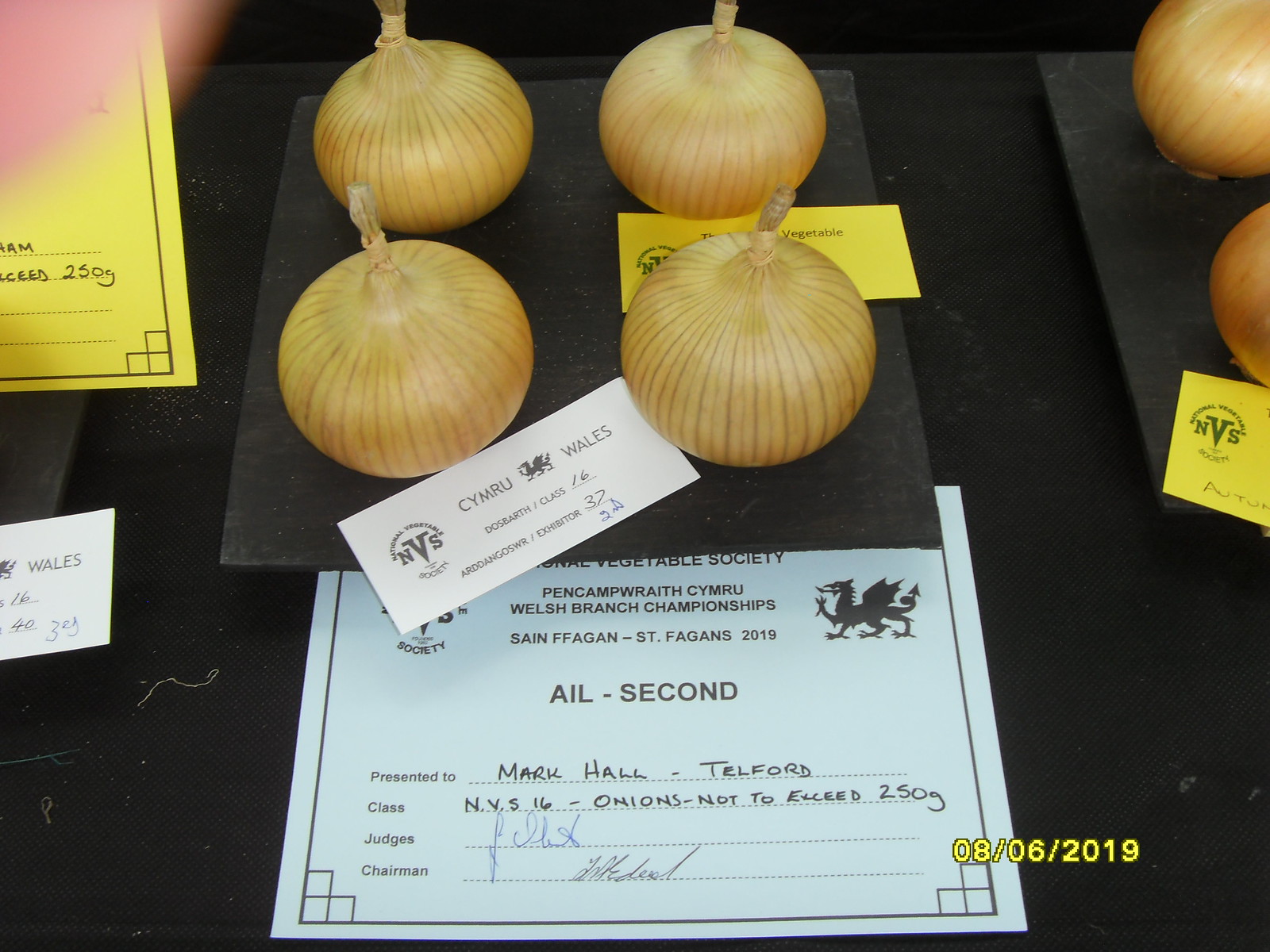This photograph captures a prize-winning entry at a vegetable society contest held on August 6th, 2019. The centerpiece of the image is a black square platter meticulously arranged with four yellow onions in a two-by-two grid. Between the two onions on the right sits a small yellow card, while a white card is positioned askew between the two lower onions. Adjacent to the platter, on the lower half of the image, is a light blue sheet delineating the award details; prominently displayed are the words "AIL-2nd" and the information that these onions, which are not to exceed 250 grams, belong to Mark Hall from Telford. Two signatures of the judges are also present. To the left and right edges of the image, partially visible, are sections of additional platters with similar arrangements of onions and yellow cards. The date "08-06-2019" is imprinted in the bottom right corner, indicating when the photograph was taken.